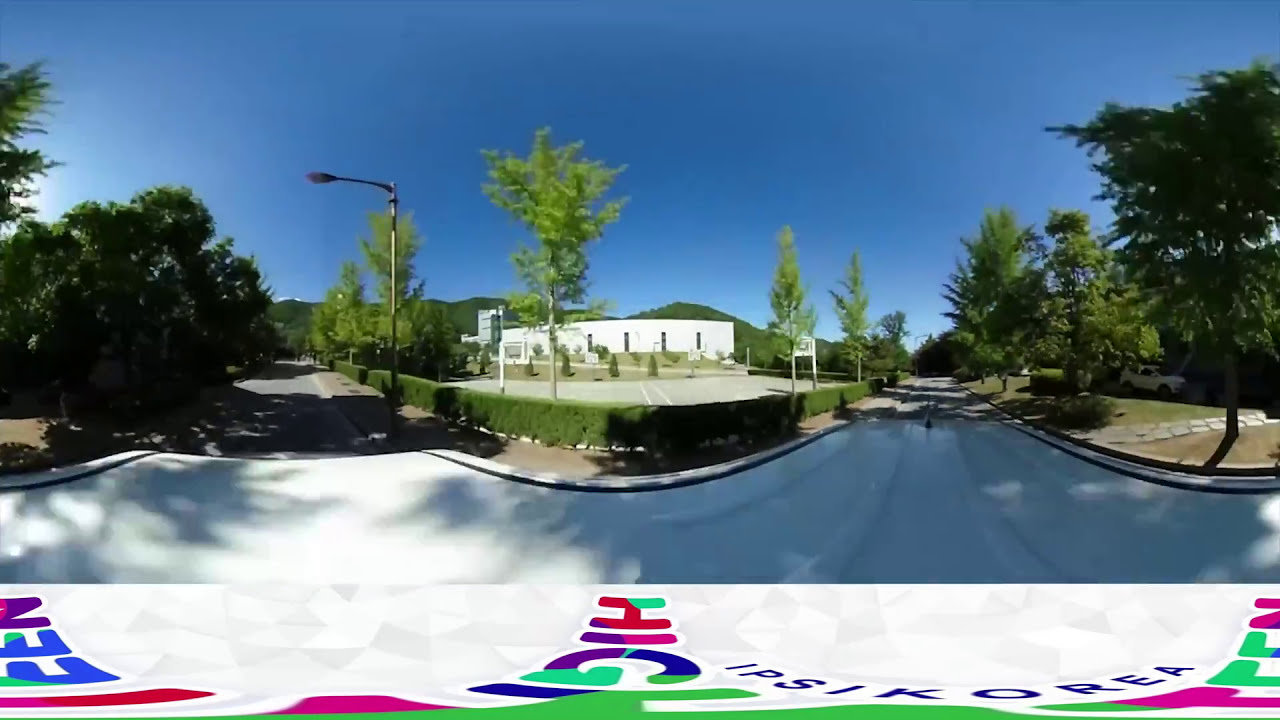The image depicts a sunny day with a clear blue sky and no clouds. At the center of the photograph stands a large, domed building characterized by its distinctive cylindrical windows. This building is surrounded by a parking lot and an abundance of green trees, enhancing the vibrancy of the setting. To the left and right of the building, two streets run parallel, each lined with green grass and tall trees, further enhancing the picturesque environment. The left street has a sidewalk adjacent to a mix of trees and bushes, whereas the right street also features a sidewalk but with more greenery on its periphery. In the background, green hills possibly covered with trees add depth to the scene. At the bottom foreground of the image, a white hood, possibly of a car or motorcycle, is visible with multicolored letters spelling out "hi" and the text "IPSI/Korea" in blue.